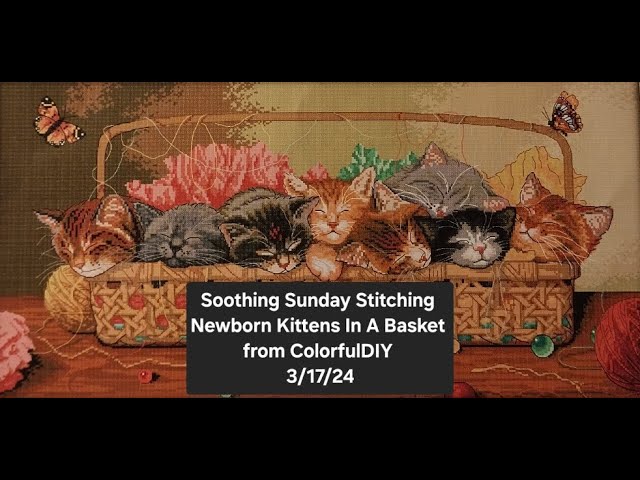The image features a detailed, cross-stitched depiction of a cozy basket filled with kittens, bordered by prominent black rectangular stripes at the top and bottom. Central to the scene is the basket containing seven tiny, snuggled newborn kittens, distributed in a pattern from left to right: an orange cat, a gray cat, a black cat, another orange cat, two more orange cats, another gray cat, and a final orange cat. These adorable kittens appear fast asleep and possess multi-colored, fluffy fur ranging from orange, gray, black, to yellow. Scattered around the basket are balls of yarn, with a prominent tan yarn ball visible outside the basket on the left. Nestled inside the basket alongside the kittens are vibrant elements that might be flowers or pillows, in hues of pink, green, and yellow. Adding a lively touch, two orange butterflies with black markings are positioned on either side of the basket, fluttering near the top left and top right. A small green marble can be seen near the lower right corner of the basket. The artwork contains text in white letters reading "Soothing Sunday Stitching Newborn Kittens in a Basket from ColorfulDIY 31724," giving it an added personal and artistic touch.